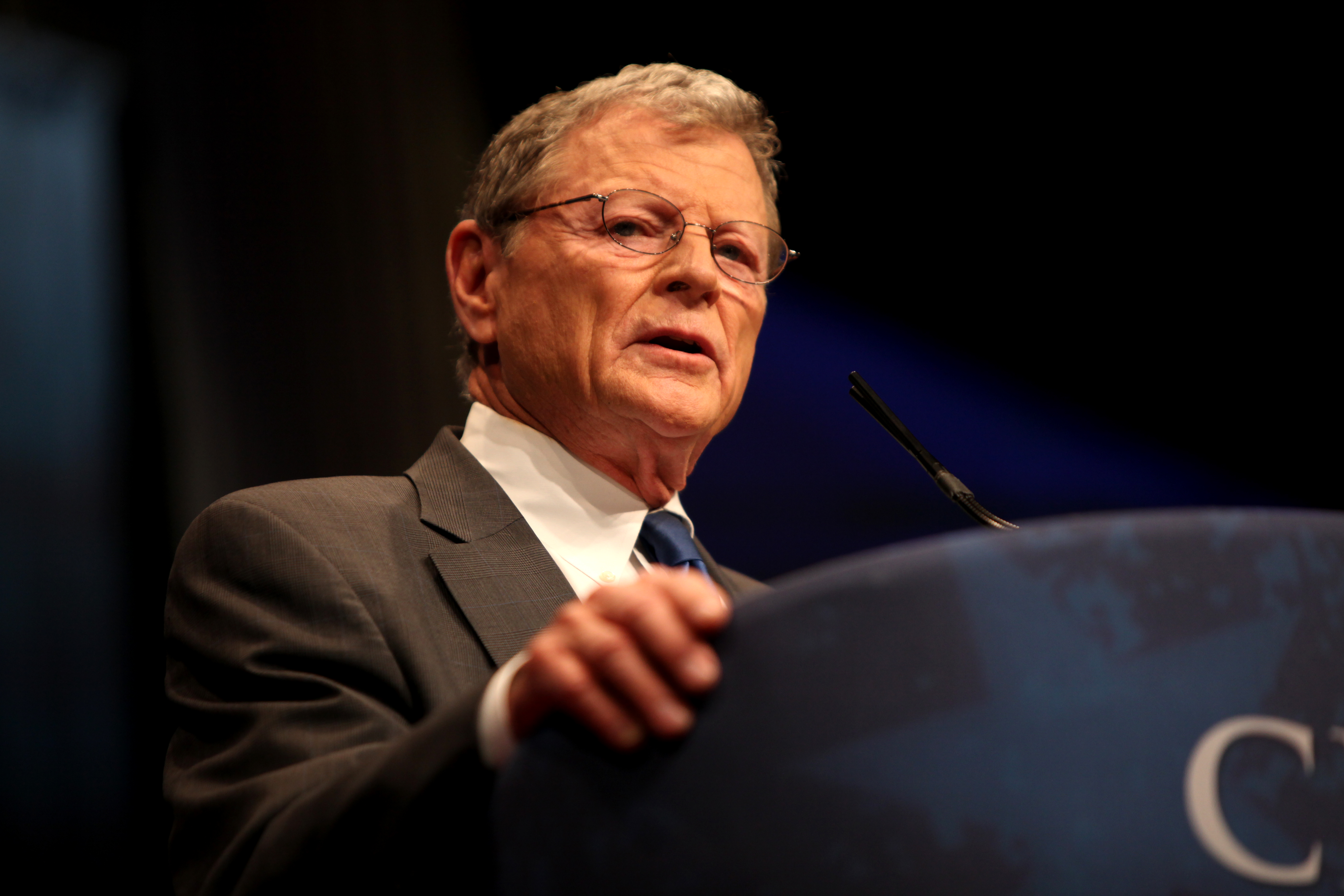In this up-close photograph taken indoors, possibly during a conference or event, a middle-aged white man is standing behind a blue and black podium, delivering a speech. The man, who has orderly parted hair that is a mixture of black and gray with more gray at the front, is dressed in a gray suit jacket, a white button-down shirt, and a blue tie. His right hand rests on the podium, and he appears to be speaking into a small, thin microphone positioned near his mouth. He is wearing thin, circular clear glasses and looks serious, gazing slightly towards the camera angle. The background features dark shades of blue and black, possibly a curtain, and has a bluish tint on the right side. The podium itself has a blue star and a partial letter "C" visible in the right-hand corner.